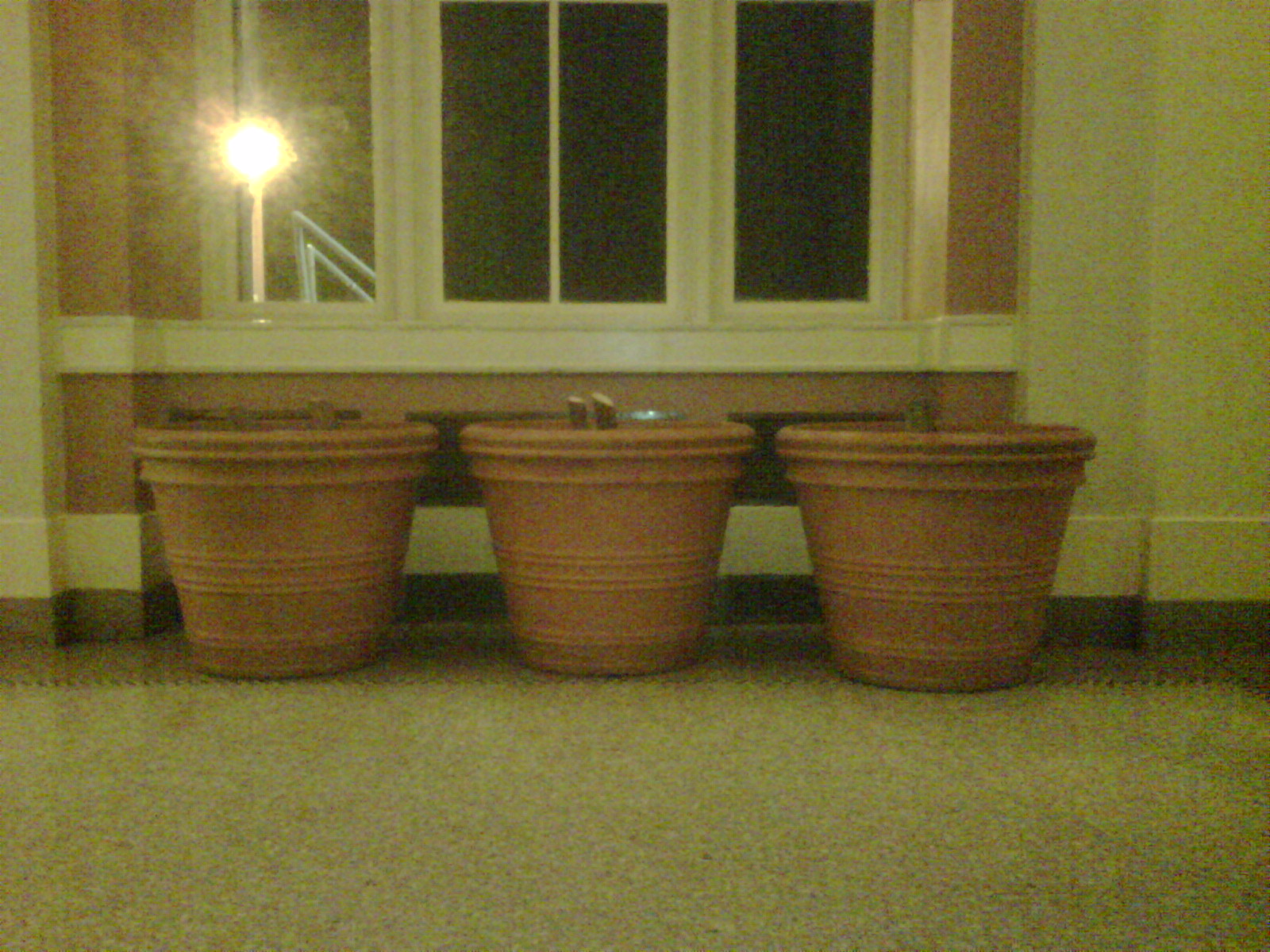This indoor nighttime photograph captures a row of three large planters positioned on a beige, short-pile rug, which sits atop wooden flooring. The planters, terracotta in color, are arranged close together with only an inch or two between them. There are no full-grown plants inside, but the middle planter has two small cut stems, and the right planter shows a hint of green emerging. The background features three tall, rectangular windows with white trims, framed by off-white walls with a slight greenish tinge from the dim lighting. The window panes predominantly show the dark night outside, with the farthest window pane revealing an outdoor light source. A bright, camera flash reflects off the leftmost window, adding a slightly pinkish glow. Despite its graininess and lack of focus, the photo offers a detailed glimpse of the indoor setting with its subtle play of textures and colors.